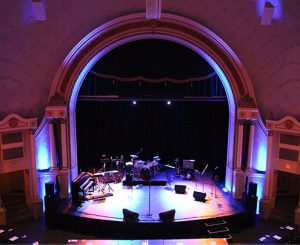In this image, we see an indoor concert hall stage set against a black background, highlighted by floodlights that create large white circles on the brown stage flooring. The stage is dominated by a large domed archway and flanked by two doors, each with a white outline; the door on the right has a red lit-up exit sign. Positioned on the stage are various musical instruments and equipment, including a drum set in the center-back, a black piano or keyboard to the left, and stacks of amplifiers, multiple microphone stands, and speakers on the right. Scattered across the stage are several black boxes, chairs, and a possible music stand. There are also ornate shelves or seating areas along either side of the stage. Steps on the bottom right facilitate access to the stage. High above, through the archway, there may be a balcony, indicating additional seating. In the foreground, a strip of rainbow-colored lights spans from dark red on the left to orange on the right, likely created by stage lighting effects that emphasize the vibrant and dynamic atmosphere of the concert hall.